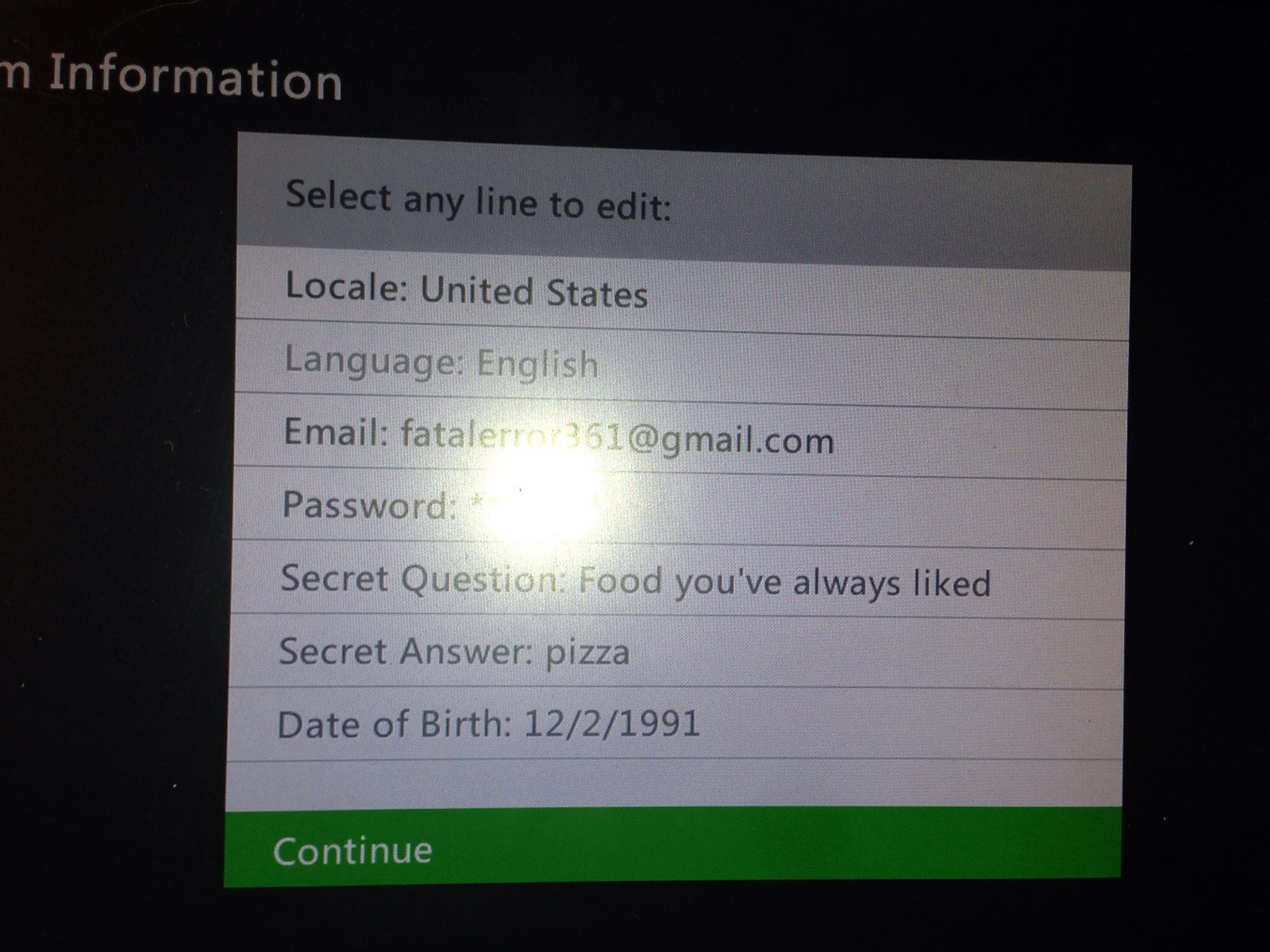The image is a photograph of a screen, likely a section of a computer or television display, showing an editing menu for a profile. On the top left corner, partially cut off, is the word "Information." The prominent part of the frame features a gray menu screen with the header, "Select any line to edit," in black text. Below this header, a series of editable fields are listed in black font on white rectangles: 

- Locale: United States
- Language: English
- Email: FatalError361@gmail.com (also referred to as badleer361@gmail.com in one description)
- Password: obscured by a single visible asterisk and a glare
- Secret Question: Food You've Always Liked
- Secret Answer: Pizza
- Date of Birth: 12/2/1991

At the bottom of the menu, a green "Continue" button is visible. The entire background of the screen is black, with a glare from the camera shining off the display, indicating that this is a photograph of the screen being taken.